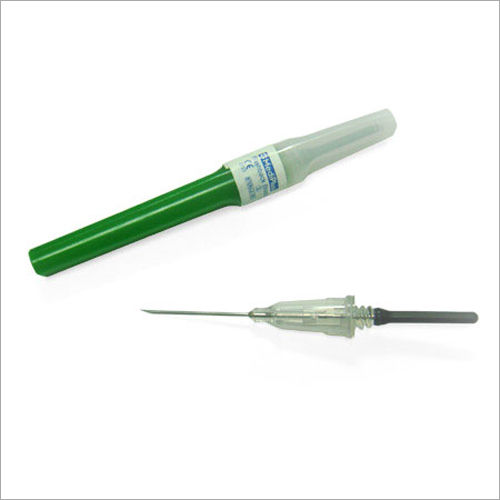The image depicts a medical device that closely resembles a green syringe, yet differs in structure. The device consists of two main components: a needle with a whitish plastic cover and a green base. Both parts are displayed on a white background. The text "MediPlus" is visible on the device in blue letters on a white section. The needle, spring-loaded and retractable, appears detached from its handle, which lies nearby. Instead of a typical syringe plunger, the contraption uses a thin piece of clear plastic around the needle, suggesting a possible alternative use, such as for collecting blood samples rather than injecting fluids. A blue and white sticker secures the top and base together, with its text remaining indistinguishable. The entire setup emphasizes a realistic photograph of the medical equipment designed for specific clinical applications.